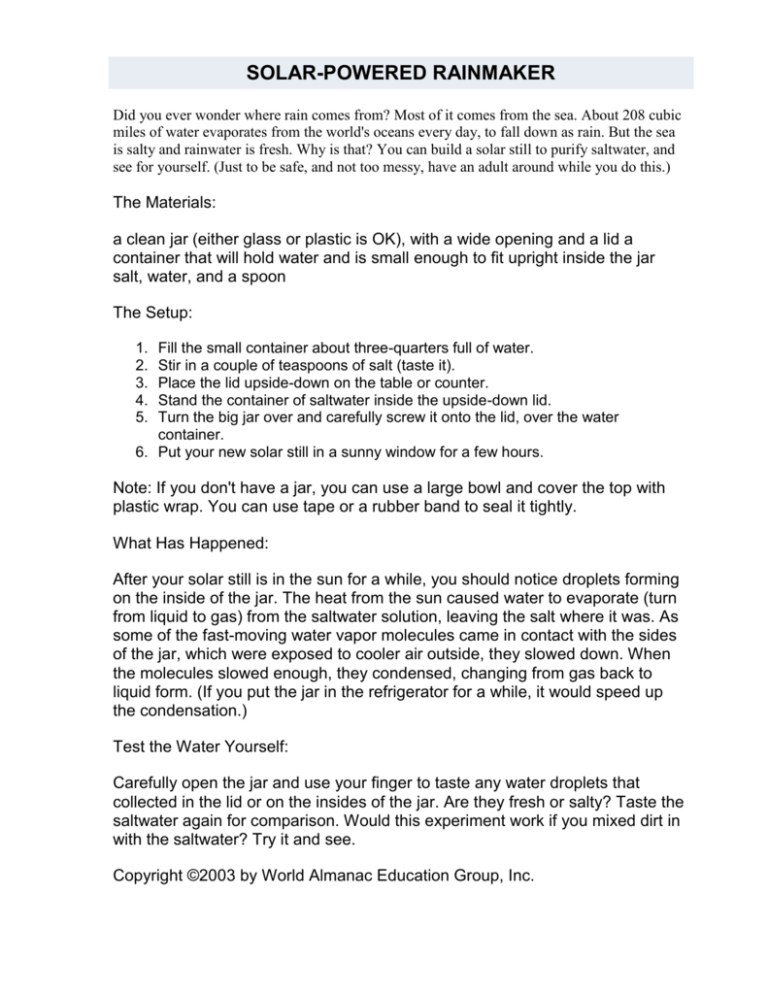**Detailed Caption:**

This image is a vertical screenshot detailing the steps and information about creating a solar-powered rainmaker. At the top of the image, there is a gray box featuring the title "Solar Powered Rainmaker" in bold, black, capital text. The contents explain the origins of rain, mentioning that most of it comes from the sea with around 208 cubic miles of water evaporating daily from the world's oceans. It highlights the distinction between salty seawater and fresh rainwater, prompting readers to explore why this happens. 

The text offers a hands-on project to build a solar stove that purifies saltwater. It advises the presence of an adult to ensure safety and avoid mess. 

**Materials Needed:**
- A clean jar (either glass or plastic with a wide opening and a lid)
- A small container that fits upright inside the jar
- Salt
- Water
- A spoon

**Instructions for Setup:**
1. Fill the small container about three-quarters full with water.
2. Stir in a couple of teaspoons of salt and taste the mixture.
3. Place the jar's lid upside down on a table or counter.
4. Stand the container of saltwater inside the inverted lid.
5. Carefully screw the big jar onto the lid over the water container.
6. Position the assembled solar still in a sunny window for several hours.

A note at the end suggests an alternative setup using a large bowl covered with plastic wrap, which can be secured with tape or a rubber band, should a jar not be available. 

The process concludes with observing the results: after some hours in the sunlight, droplets will form on the inside of the jar, illustrating the principle of solar distillation.